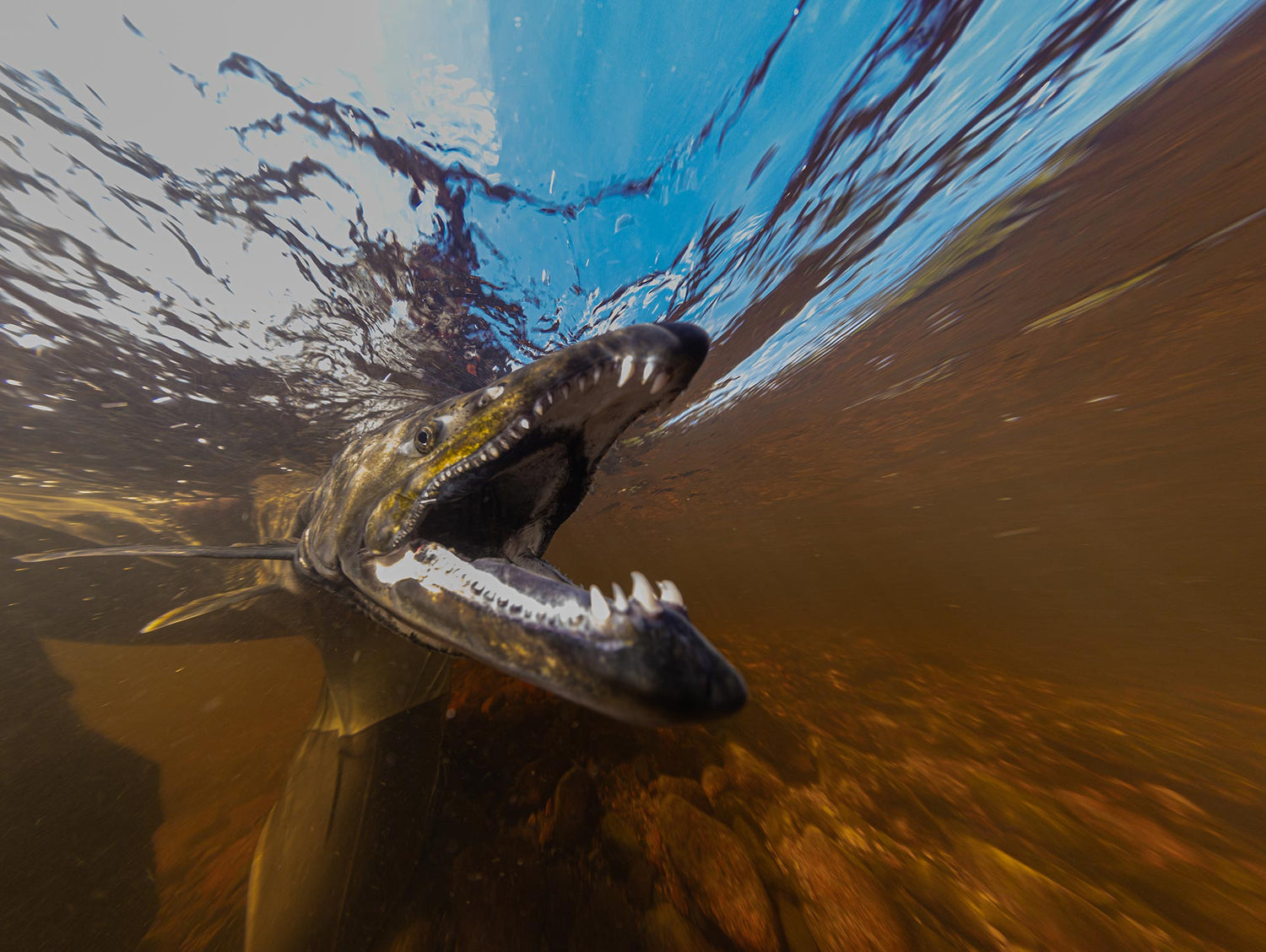This detailed underwater photograph captures a striking fish, possibly a gark or a barracuda, positioned centrally and taken with a wide-angle, fish-eye lens. The fish is swimming in shallow, murky water, close enough to the surface that the wavy reflection and refracted light reveal a blue sky above, contrasting with brownish hues on the right side of the water. The fish's defining features include a long snout and an array of jagged, serrated teeth, with the largest ones prominent in the upper and lower front of its jaw, surrounded by spiked teeth encompassing the rest of its mouth, which is wide open, suggesting it is about to catch some prey. The creature has a dark gray body with subtle yellow accents around its mouth, and a barely visible fin on the left-hand side. Interestingly, behind the fish, part of a person can be discerned, with one leg straight and the other bent, possibly in the act of releasing the fish into the water. Despite the detailed view of the fish's head and mouth, its tail and other body parts remain out of sight, emphasizing the sheer scale of its gaping maw.